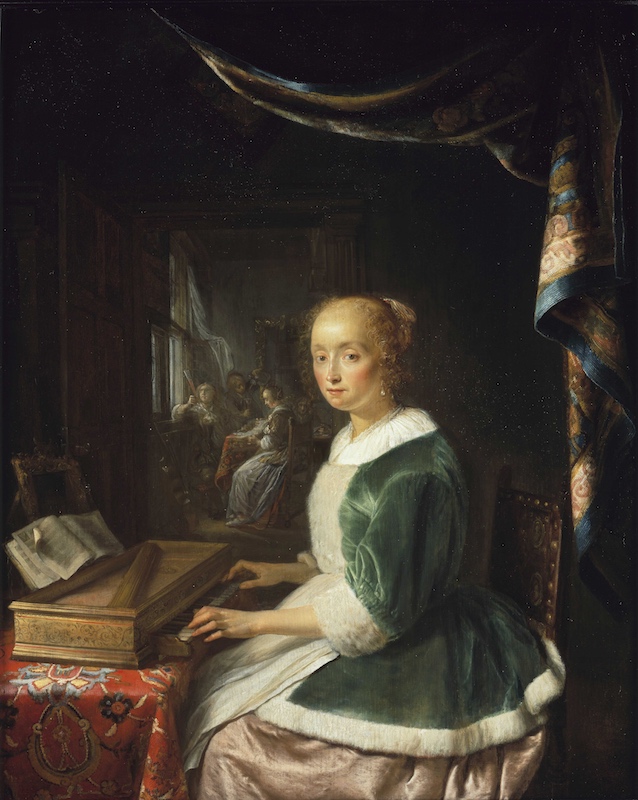The painting depicts a woman from an earlier era, possibly the 1700s, playing a piano. She is wearing an elegant green top, resembling a velvet coat with white frills and cuffs that reach her elbows. Her attire is complemented by a pinkish, purple skirt. The woman’s blonde hair is pulled back into a bun, and her cheeks are slightly flushed. Both of her hands rest on the piano keys, which are part of a wooden piano positioned on a table with a red oriental-patterned tablecloth. An open book lies on the piano, suggesting she is reading music. She gazes directly at the viewer. In the dimly lit background, there are three figures, likely women, seated by a window with a faint light illuminating them. Above and to the right of the woman, there is a luxurious drape featuring hues of blue, pink, and orange.